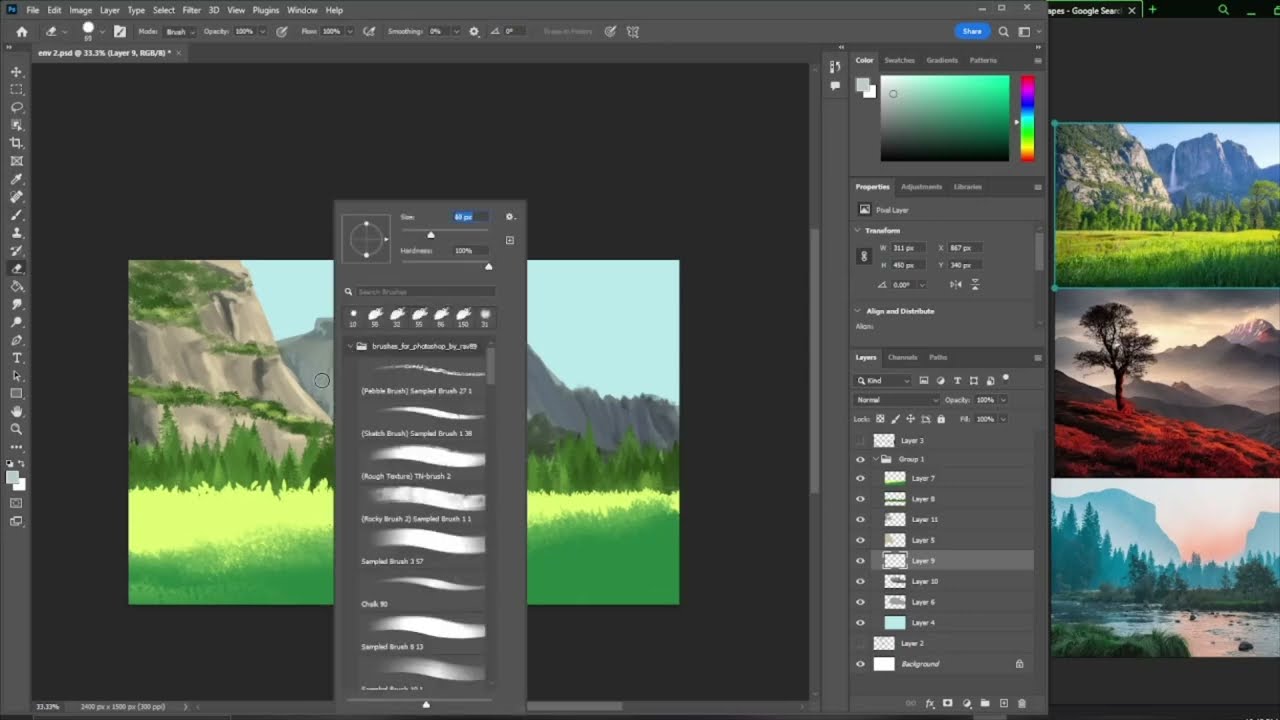This image is a detailed screenshot of a computer screen showcasing an image editing process in the Photoshop application, identifiable by its distinct logos and interface elements. The screen is set in night mode, displaying a dark gray and black background. On the left side, a painted nature scene is being manipulated, featuring hills, trees, mountains, and waterfalls, with a meadow of green grass and cliffs behind it. A large gray box shows various brush stroke options, visible through a menu dropdown, and a color spectrum field with blue, green, and rainbow hues for color adjustments. On the right side of the screen, three vertically stacked nature photographs serve as references or layers within the Photoshop dialog box. The top photo depicts a green field with cliffs, the middle one presents a red field with black mountainous silhouettes and fog, and the bottom photo shows a river flanked by grass and trees with blue mountain silhouettes and a red sky. The detailed layers and editing tools underscore the user's focus on enhancing the realism of the nature scenes, possibly converting them into more cartoonish versions.